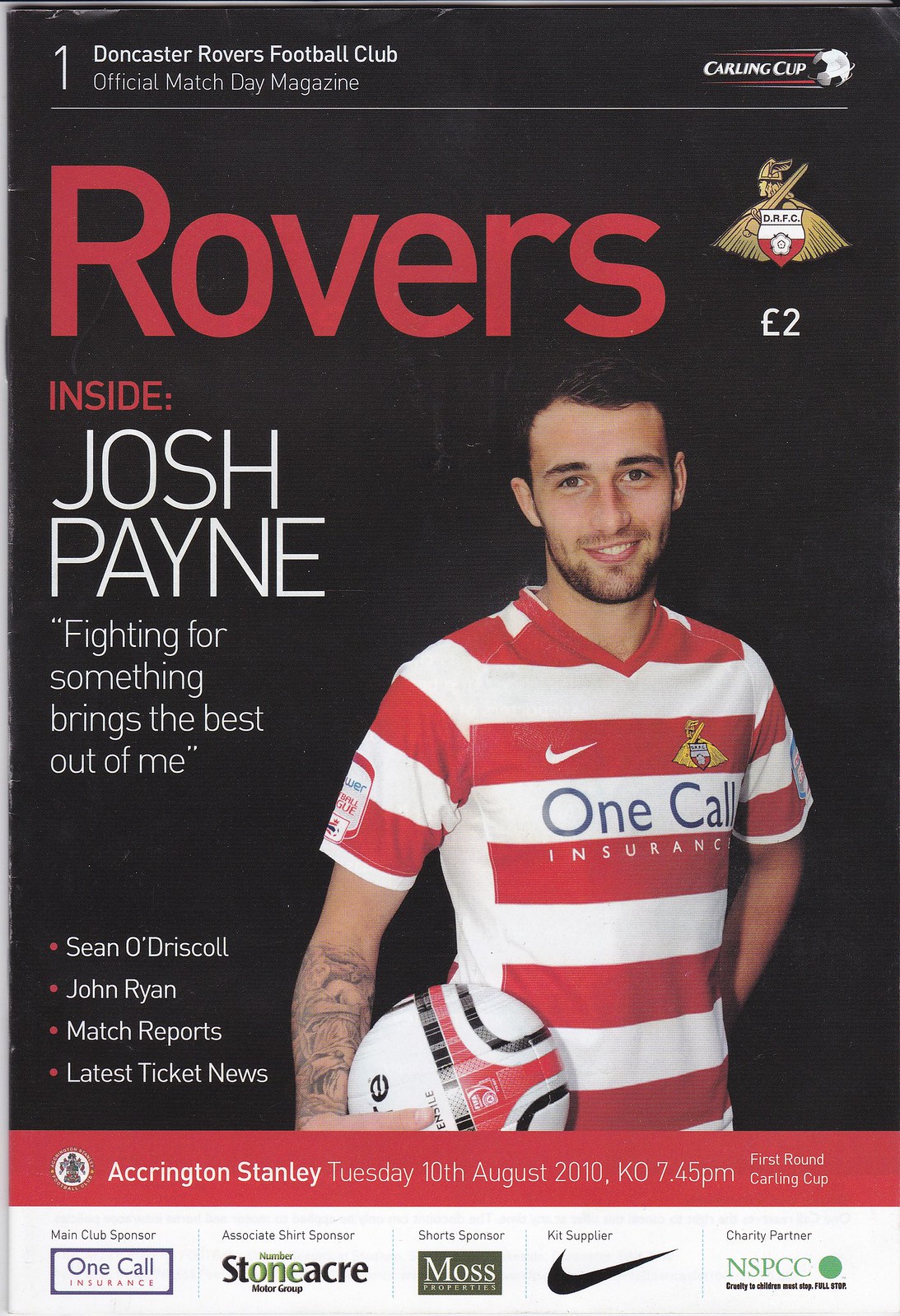This image depicts the front cover of the Doncaster Rovers Football Club Official Match Day Magazine. Prominently featured is a man smiling at the camera while holding a soccer ball against his hip with his right hand. He is wearing a short-sleeved red and white striped shirt adorned with a Nike logo on the left side of the chest and another insignia on the right. The shirt also displays the text "One Call Insurance" in black. The club's logo—a gold Viking with a winged metal helmet, a sword over his shoulder, and a shield with the letters "DRFC"—is present on the cover as well.

At the top of the cover, the text reads, "Doncaster Rovers Football Club Official Match Day Magazine" in white letters. To the right of this, it says "Carling Cup." Below, in bold red letters, is the word "ROVERS." Beneath this, more details include the headline, "Inside Josh Payne—Fighting for Something Brings the Best Out of Me." Additional captions include mentions of other features: "Sean O'Driscoll," "John Ryan," "Match Reports," "Latest News," and "Latest Ticket News." The issue also notes an event: "Accrington Stanley Tuesday 10th August 2010 Kickoff 7:45." The bottom of the page features a red trim.